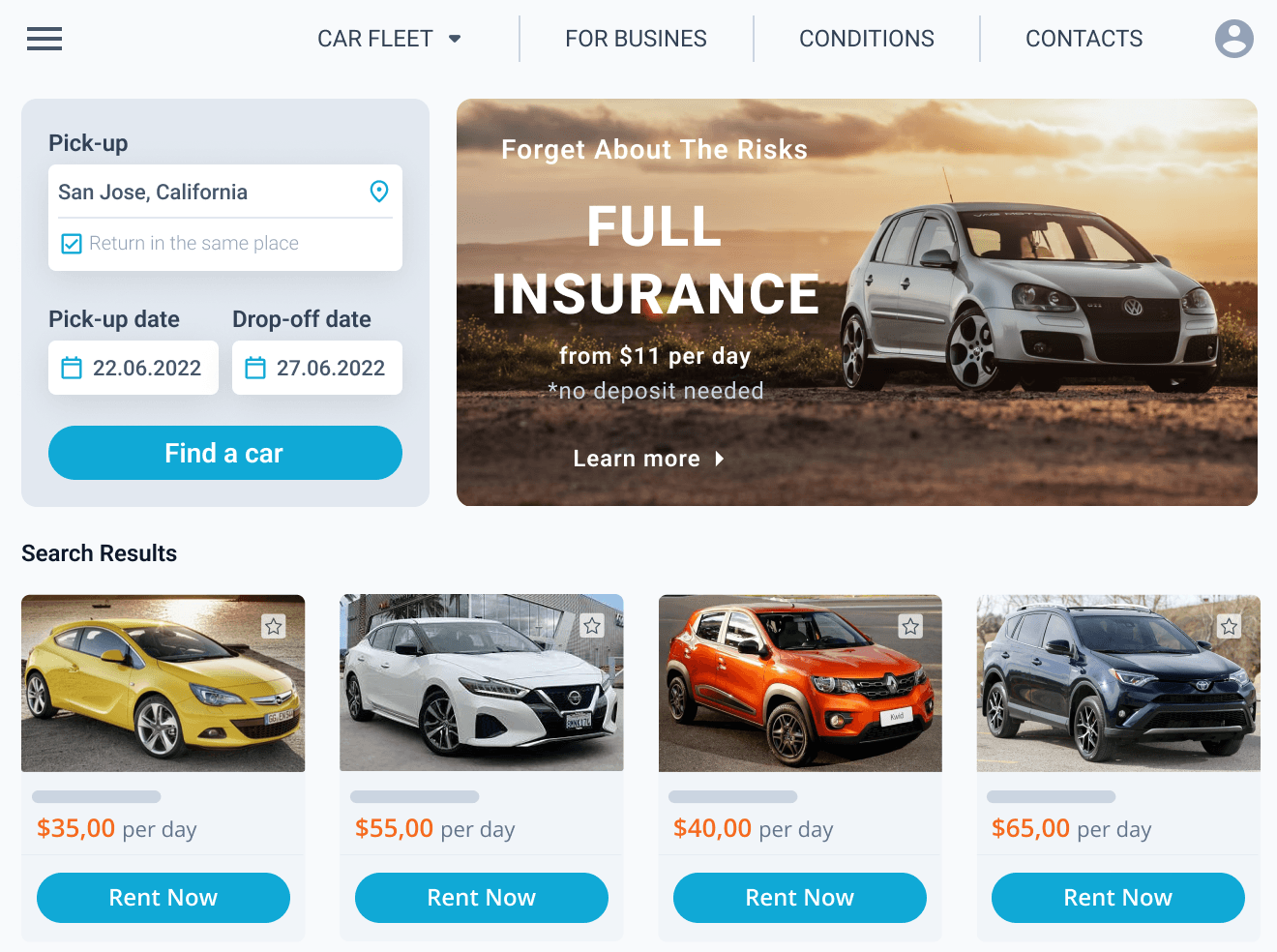The image depicts a car rental website interface. On the left-hand side, there is a navigation menu icon represented by three horizontal lines stacked vertically, commonly known as the hamburger menu. Adjacent to the menu icon is the label "Car Fleet" with a dropdown menu featuring options such as "Business," "Conditions," and "Contact." To the right, there's a circular icon with a person silhouette, presumably for user account access.

Below these icons, the interface has fields for picking up and dropping off the rental car. The "Pick Up" location is set to "San Jose, California," with a checkbox indicating the car should be returned to the same location. The pick-up date is listed as "02.06.2022," and the drop-off date is "27.06.2022." A prominent blue button labeled "Find a Car" is located to the right of these fields.

The website highlights an insurance option with the text, "Forget about the risks! Full insurance from $11 per day* No deposit needed." There is an arrow pointing to additional information. A background image shows a car against a landscape with a sun, clouds, and hills.

The page also displays search results for rental cars:
1. A yellow car available for $35 per day, with a blue "Rent Now" button.
2. A white car mistakenly listed for $5,500 per day, also with a blue "Rent Now" button.
3. A red car priced at $40 per day, featuring a blue "Rent Now" button.
4. A car in black or midnight blue, available for $85 per day, accompanied by a blue "Rent Now" button. 

Each blue "Rent Now" button is styled with white font.